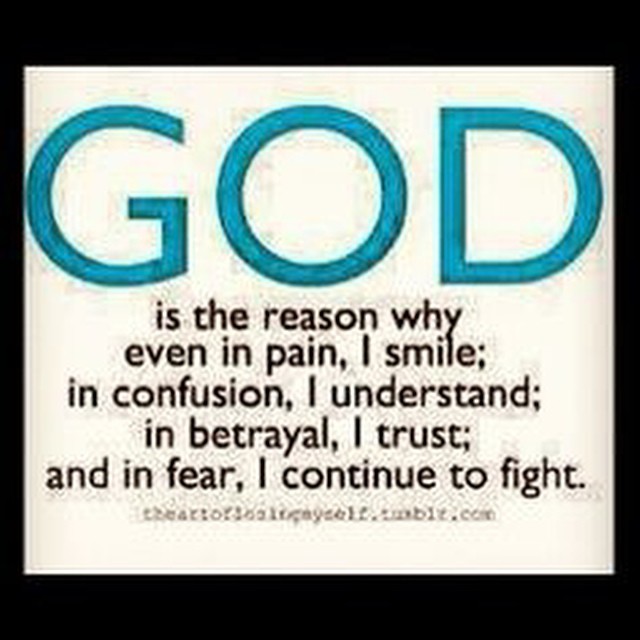This image is a low-quality graphic that you might typically find shared on social media. It features a white square set against a black background. At the top of the square, in large aqua blue letters, is the word "G.O.D." Below this, in smaller black text, is an inspirational quote that reads: "G.O.D. is the reason why even in pain I smile; in confusion I understand; in betrayal I trust; and in fear I continue to fight." The text is pixelated, making it appear somewhat blurry. At the bottom of the square, there is a website URL for a Tumblr blog titled "theartofsomethingmyself.tumblr.com." This graphic has a motivational and religious tone, commonly found in posts shared for encouragement and inspiration.